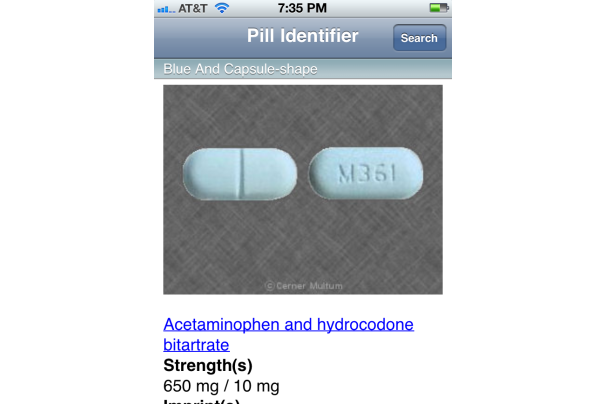The image is a screenshot from a smartphone displaying various details from a pill identification app. 

At the top left corner of the screen, the AT&T network provider is shown, with the current time, 7:35 PM, displayed in the center. The battery icon on the top right indicates a half-charged battery. These elements are set against a gray background.

Below this, the app interface begins with a dark gray backdrop, featuring the title "Pill Identifier" in white text. Underneath, a prominent dark blue button labeled "Search" in white text is visible.

Further down, another section with a gray background contains the text "blue and capsule-shape" in white. This is followed by an image depicting an oblong, white pill with a dividing line in the middle and the imprint "M361" on the right side.

Beneath the pill image, the copyright notice "Copyright Cerner Motum" is displayed, followed by a blue hyperlink reading "acetaminophen and hydrocodone bitartrate." 

The bottom portion of the screen details the pill’s strength in bold black text labeled "Strength (S)." Below this label, the specific dosage is listed in non-bold black text as "650 milligram / 10 milligram."